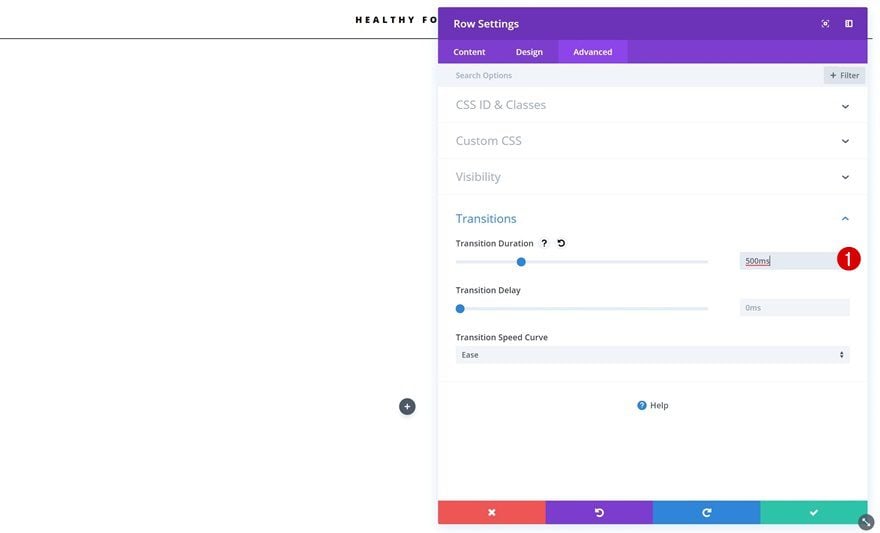A screenshot captures the interface of the Divi Visual Page Builder, a well-known WordPress theme, specifically focusing on the 'Row Settings' section within the design editor. At the top of the interface, a purple bar displays the title 'Row Settings,' accompanied by a gear icon for settings on the far right. Below this title bar, three tabs labeled 'Content,' 'Design,' and 'Advanced' are present, with the 'Advanced' tab currently selected.

Within the advanced settings panel, there are several options categorized under different headings: 'Search Options,' 'CSS ID and Classes,' 'Custom CSS,' 'Visibility,' and 'Transitions.' The transitions section allows users to configure the transition settings with a duration slider set to 500 milliseconds, a transition delay (currently unset), and a transition speed curve set to 'Ease.' Below these settings, a help section provides additional guidance.

At the bottom of the panel, a red 'X' for canceling changes is visible alongside green, purple, blue, and orange icons, which likely represent actions such as saving changes, applying presets, and accessing more options. On the left side of the screen, a plus icon within a circle suggests functionality for adding new elements or rows to the page.